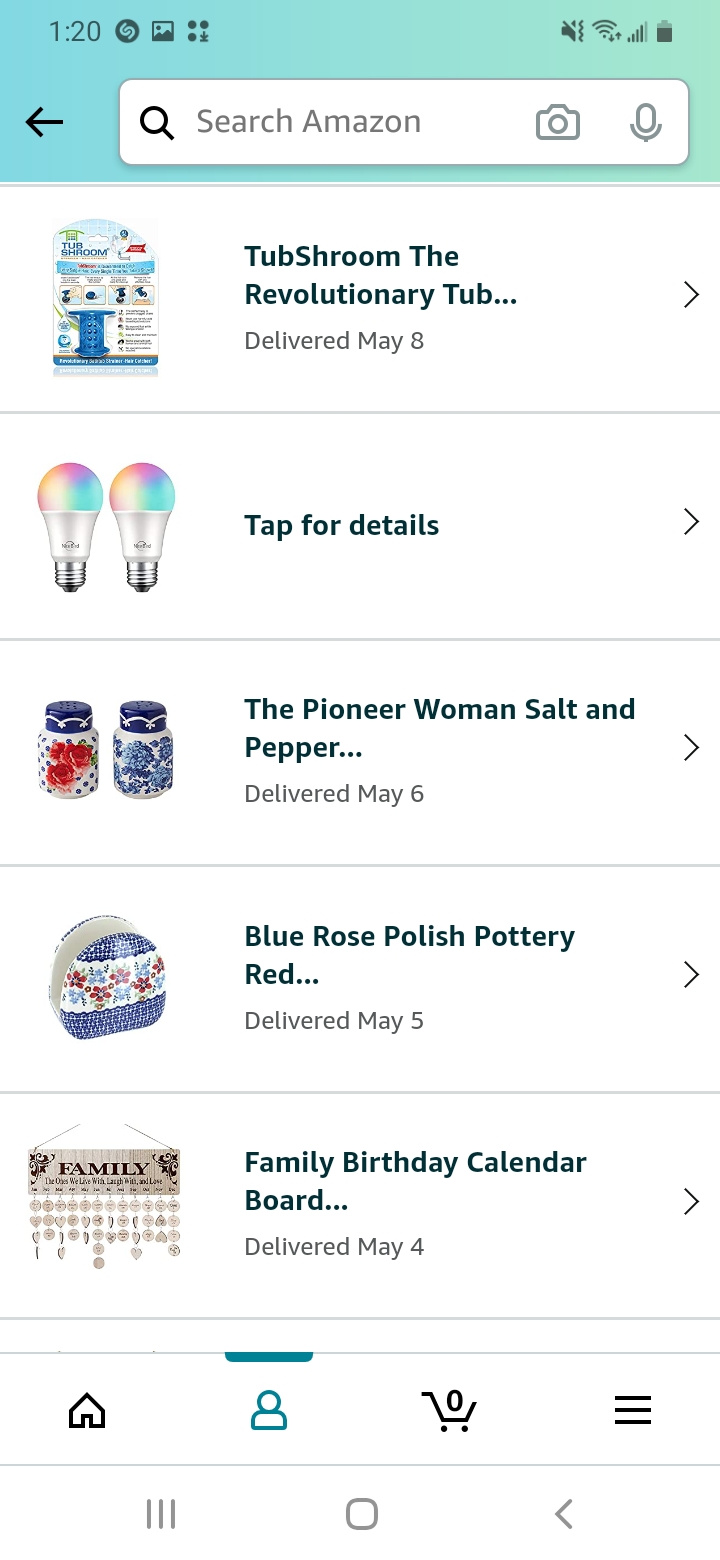**Detailed Caption:**

A screenshot captures a smartphone displaying the Amazon app. At the top of the screen, a turquoise header bar features a central white search bar that includes the text "Search Amazon" in gray, accompanied by a gray magnifying glass, a photo icon, and a microphone icon within the search box. 

Below the header, the screen is organized into a single column listing various products that have been ordered through the user's Amazon account. Each product entry starts with a photo on the left side, followed by the product name and, in some cases, a delivery date on the right. A gray right-facing arrow (caret) appears next to the product information, and each entry is distinctively separated by a horizontal gray line.

The listed products include:

1. **TubShroom, The Revolutionary Tub** - A bath accessory depicted in its image.
2. **Tap for Details** - Accompanied by two light bulbs, suggesting more information is available.
3. **The Pioneer Woman Salt and Pepper** - A pair of candles with a note stating "Delivered May 6th."
4. **Blue Rose Polish Pottery Red** - Displaying an image of pottery, though the specific item is partially obscured in the text.
5. **Family Birthday Calendar Board** - Featuring an image of a birthday calendar board.

The clean and systematic presentation allows for easy browsing and management of previously ordered items.